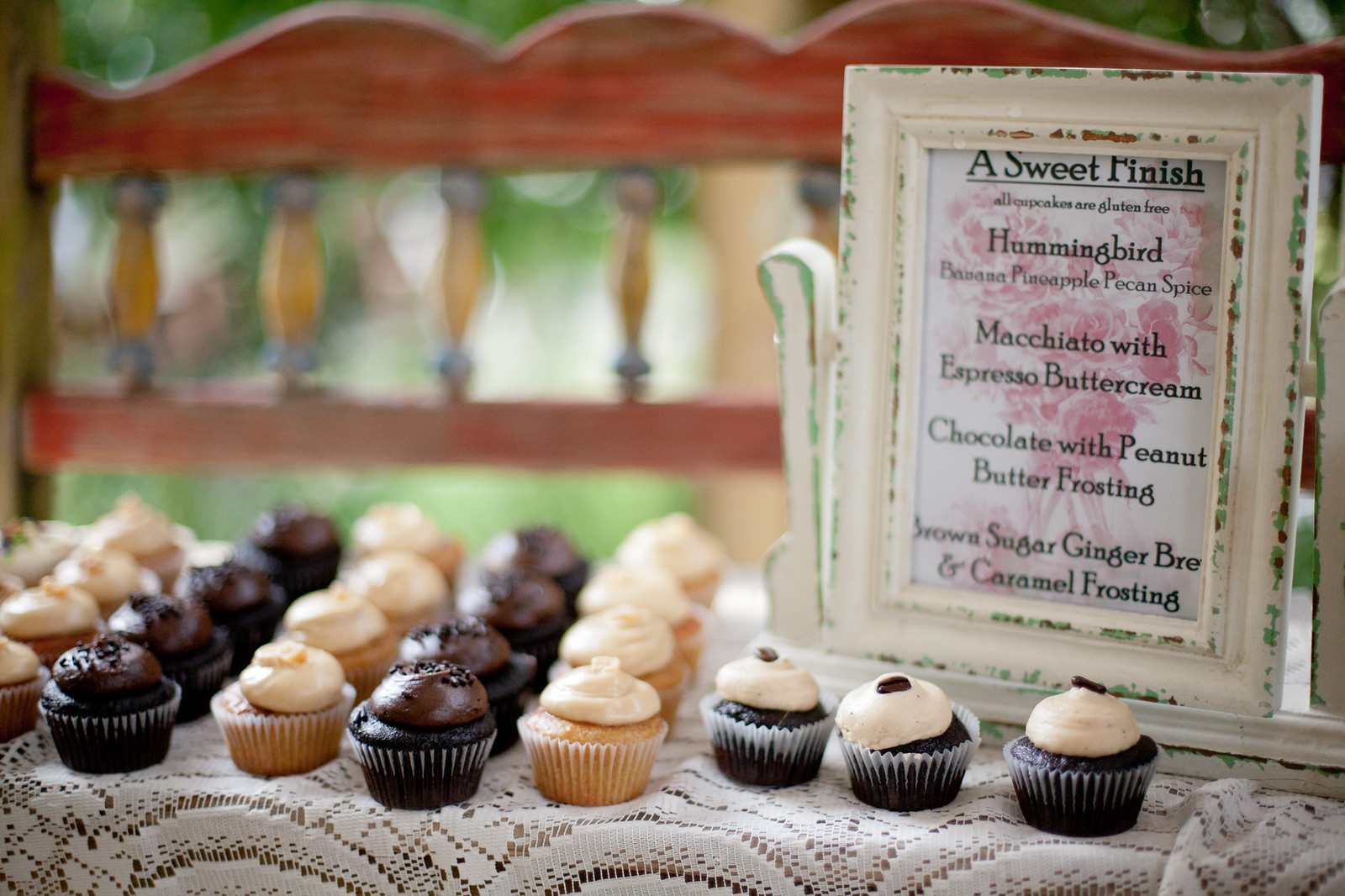The image depicts a table adorned with a white lacy tablecloth, displaying rows of miniature cupcakes. These cupcakes are arranged in four deep rows, with the ones at the front in sharp focus, gradually becoming blurry towards the back. There are alternations of chocolate cupcakes and tan vanilla cupcakes. The chocolate cupcakes feature either chocolate frosting, vanilla frosting with a black dot, or vanilla dollops. Meanwhile, the vanilla cupcakes are topped with vanilla dollops. All the cupcakes are in disposable wrappers. To the right of the display, there's a framed sign that reads "A Sweet Finish" and lists the cupcake flavors: hummingbird, banana, pineapple, pecan spice, macchiato with espresso buttercream, chocolate with peanut butter frosting, and brown sugar gingerbread with caramel frosting, all of which are gluten-free. In the blurry background, a bench and some trees are faintly visible, providing a serene outdoor setting for the detailed and appetizing cupcake arrangement.